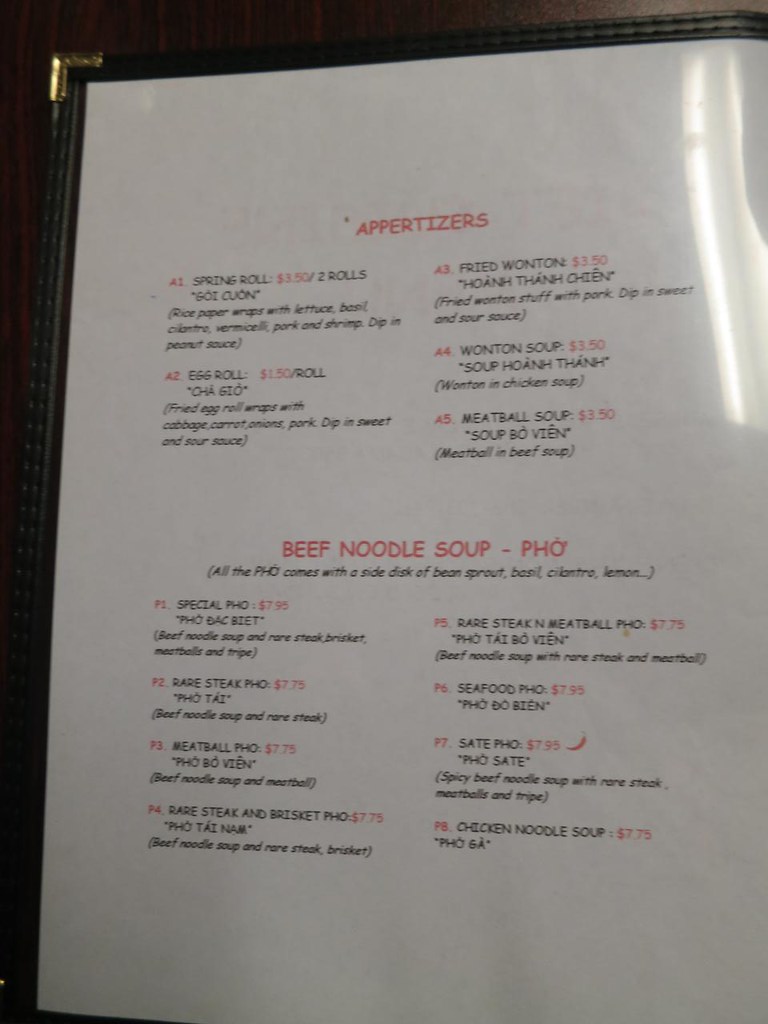A detailed photograph showcases a menu page encased in a protective plastic sleeve, housed within a sophisticated leather-bound book. The right side of the menu page features a soft reflection of fluorescent lights. The page itself is white, boasting a visible paper texture. The left page of this booklet prominently displays the section header "Appetizers" in striking red text at the top. Beneath this header, there are five distinct items, listed in two columns. 

In the left column, the items are:
1. Spring Rolls
2. Egg Rolls

In the right column, the items are:
1. Fried Wonton
2. Wonton Soup
3. Meatball Soup

Each item name is written in black text, followed by detailed descriptions in Vietnamese, with the prices highlighted in red.

The bottom half of the page is dedicated to "Beef Noodle Soup, Pho," labeled in red. This section contains eight items, listed in two columns as follows:

In the left column, the items are:
1. Special Pho
2. Rare Steak Pho
3. Meatball Pho
4. Rare Steak and Brisket Pho

In the right column, the items are:
1. Rare Steak and Meatball Pho
2. Seafood Pho
3. Satay Pho
4. Chicken Noodle Soup

Similar to the appetizers, each item here is listed in black text with detailed descriptions in Vietnamese underneath, and the prices are displayed in red on the right. The meticulous arrangement ensures clarity, making the menu both informative and visually appealing.